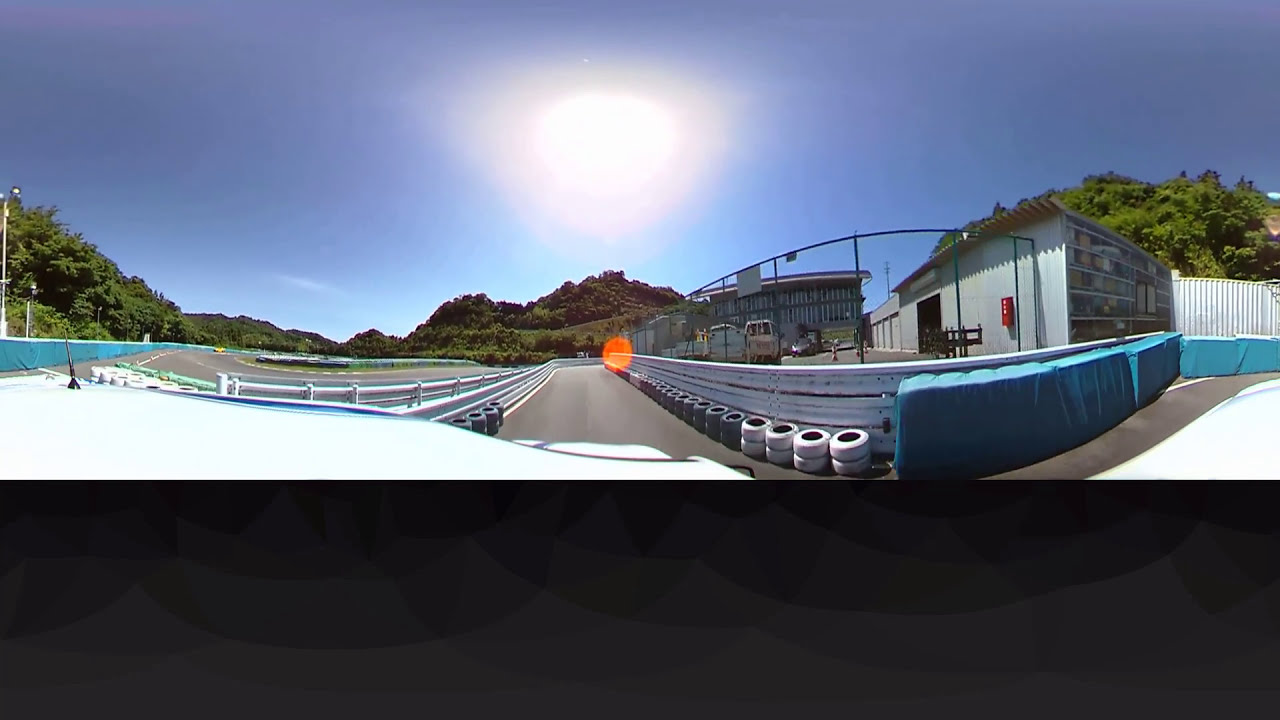This is a horizontally aligned rectangular photograph capturing a sunny, cloudless day with a clear blue sky and a bright white sun positioned at the center. Below the sky, a large hill or mountain, characterized by brown rocky sides and dense green tree coverage, stretches across the scene, flanked by additional clusters of trees on both the far left and right sides. 

In the middle of the image, there appears to be a paved racetrack marked by a distinctive blue wall along its perimeter, which is likely padded. A yellow sports car can be distinguished in the distance along the track, which curves and features railings. On the right side, several tires are lined up against a white wall, adjacent to more sections of the blue wall. Further right, a grey building with a corrugated metal roof and a large black chain-link fence can be seen. The building has an open garage door in its center and a red box affixed to its exterior. In front of it, several vehicles, likely white vans, are visible.

The bottom portion of the picture contains a horizontal black and gray rectangle, creating a visual disconnect from the rest of the bright and detailed outdoor scene.